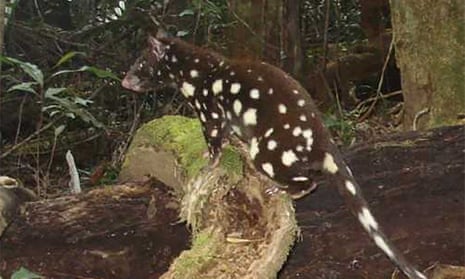In a dense woodland setting, a large, furry rat-like creature with a pointy face and small ears sits alert on top of a fallen, moss-covered log. Its dark brown coat is speckled with bright white splotches, and its long tail hangs down towards the right corner of the image. The log, intertwined with a root covered in fungus, extends into a lush background filled with vibrant vegetation, trees, and heavy foliage. Two tree trunks are visible at the top right, while the left side features thick greenery that continues deep into the forest. The rat, with a pink nose, appears ready to pounce, fixating its gaze to the left.